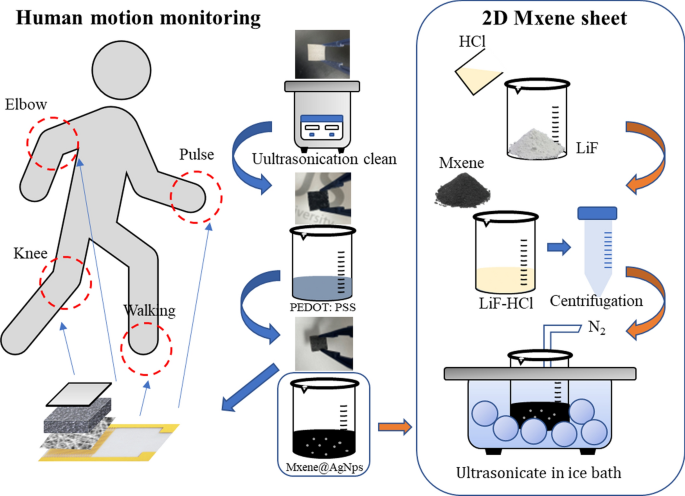The image resembles a detailed diagram from a science textbook. It prominently features a 2D illustration of a human figure at the top left, labeled "human motion monitoring." This figure is gray with a black outline and has red dashed circles around various joints, including the elbow, knee, and foot. Below these joints, there are annotations and a sequence of small squares representing different motion data.

Adjacent to this human figure, there is a vertical stacking arrangement of beakers labeled "ultrasonication clean." The diagram details multiple stages of scientific processing, with each beaker containing different substances. One beaker is marked "PEDOT;PSS," while the others display labels like "2D Maxine Sheet HCI" and "ultrasonicate in ice bath," depicting different stages and treatments. The beakers contain substances of various appearances, including grainy white material and black grains.

To the right of this, there's a detailed layout describing the "2D Maxine Sheet" procedure, featuring beakers and arrows pointing to each stage of the process, which includes ultrasonication and incubation steps. Arrows connect the beakers and point towards annotations and the human figure, illustrating the scientific method and its application to human motion monitoring.